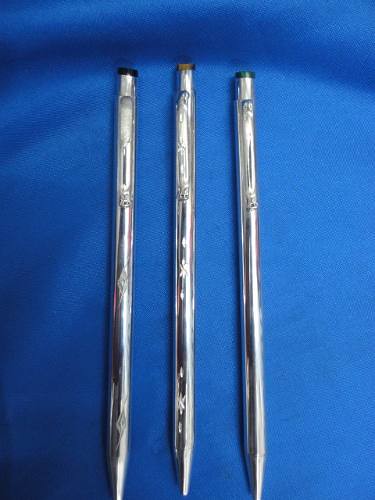This detailed photograph showcases three elegant silver pens meticulously arranged on a striking teal blue silk handkerchief, serving as a luxurious backdrop. The pens are aligned vertically in parallel, presenting a professional and staged appearance. Each pen features a distinctive colored cap top, with the left pen sporting a black top, the central pen adorned with an amber gold top, and the right pen crowned with a green top. The pens exhibit sleek designs running from the tops down to their pointed tips. They are characterized by their shiny, reflective surfaces and are equipped with clips for attaching to clothing or accessories. The pens' twist mechanisms are subtly highlighted, adding functional sophistication to their aesthetic appeal. Though there are intricate engravings on each pen, the fine details remain elusive due to the small size of the markings.